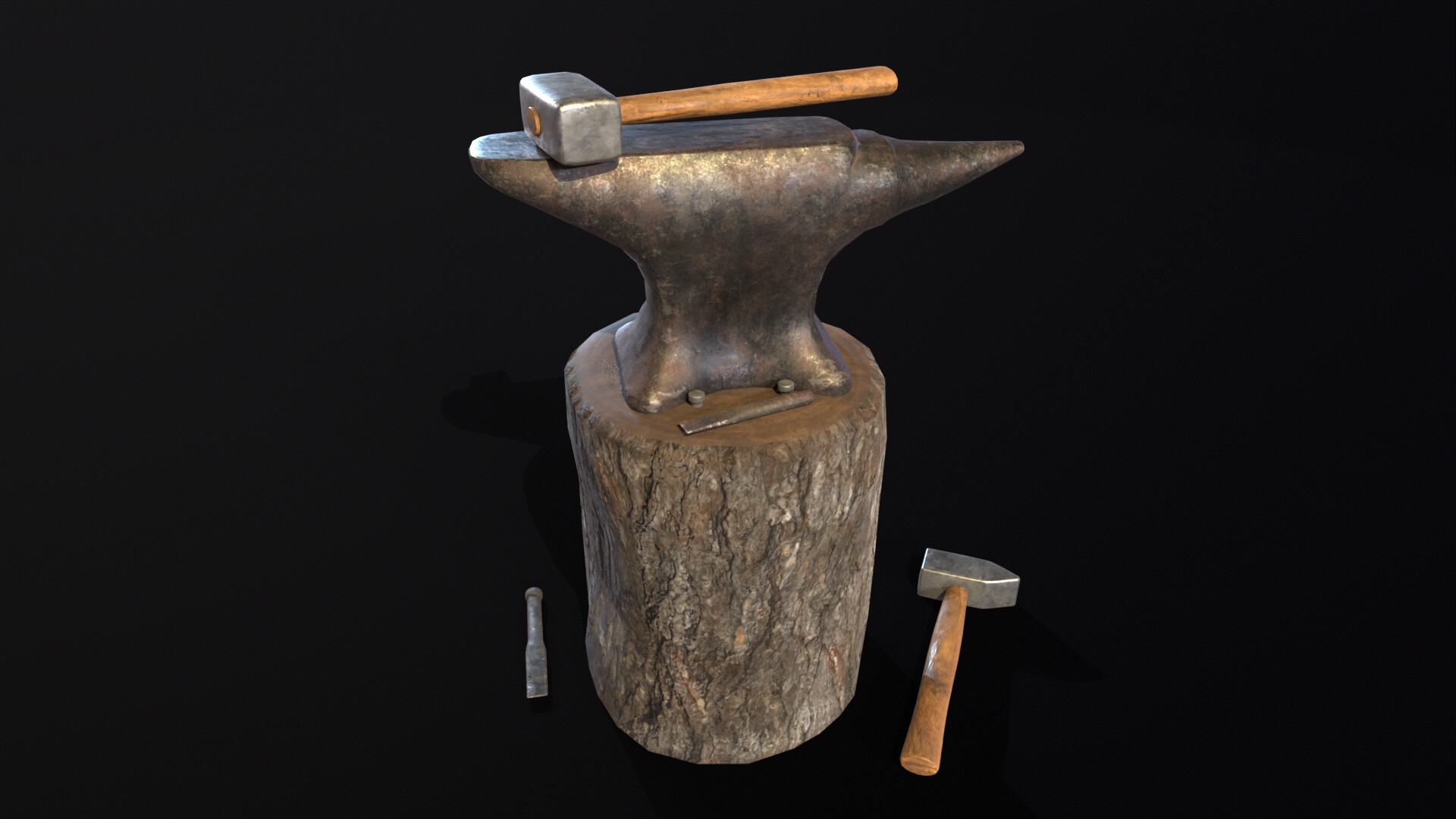This 3D rendering depicts a detailed blacksmith's anvil setup. At the center is a large, typical blacksmith anvil with a flat surface on top, a pointed horn on the right end, and a curved, rounded heel. The anvil is securely mounted with multiple bolts onto a sturdy, cut log with a smooth, flat top and rough, bark-covered sides. On the anvil's surface lies a substantial rectangular-headed hammer with a light brown wooden handle. To the right of the stump, there's another hammer, characterized by one flat side and a triangular point on the other. Adjacent to this hammer is a metal rod chisel with a slightly pointed, flat end. Another similar chisel is positioned on the top surface of the log next to the anvil. The entire scene is set against a solid black background, highlighting the detailed textures and forms of the tools and the log.